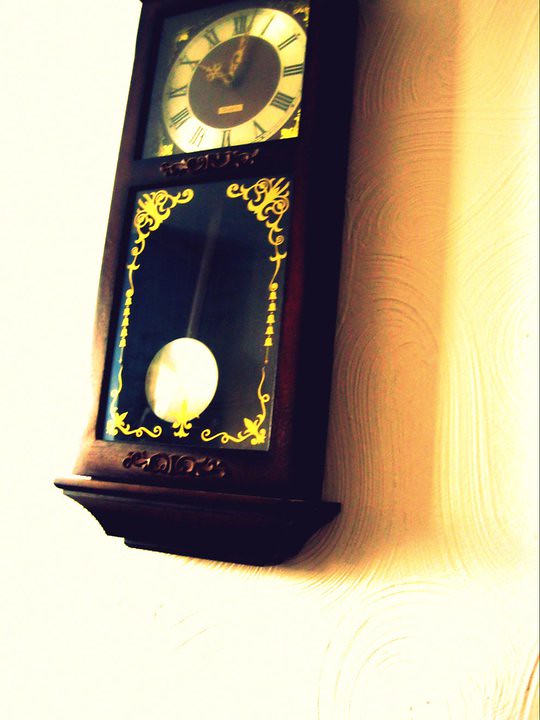This image showcases a intricately detailed miniature grandfather clock mounted on a plastered wall. The wall features an old-school design with visible swirls in a white pattern. The clock is viewed from a close-up, side-angle, and slightly underneath, capturing the entirety of its elegant structure. The clock's face exhibits Roman numerals in black, enclosed by a bronze-colored outer ring and a brown inner circle. The hands of the clock are also bronze, pointing to the time of 10:02. Below the clock face is a visible pendulum with a bronze medallion, encased in a structure embellished with gold-plated designs. The clock appears in two distinct parts against the intricately patterned white plaster wall, creating a striking contrast between the antique timepiece and the ornate backdrop.